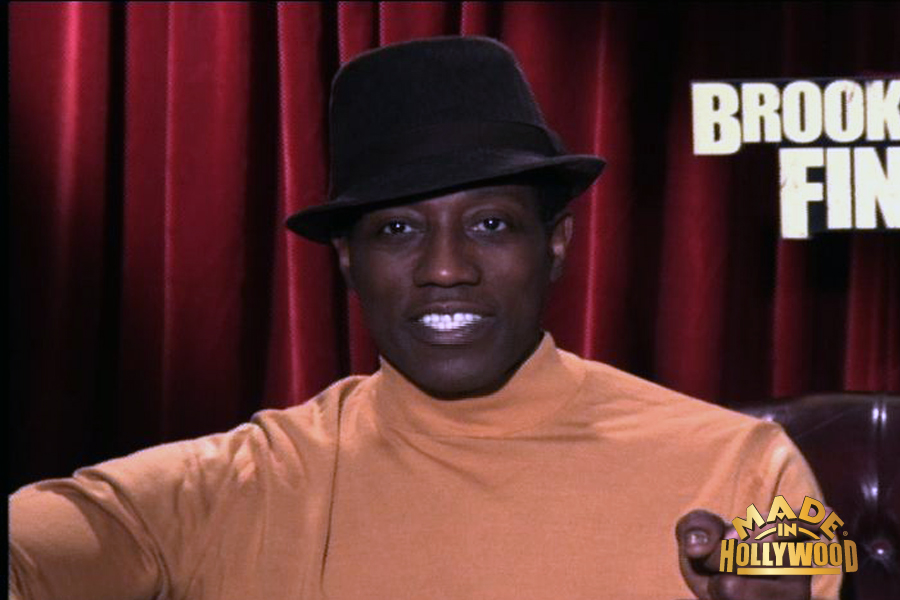The image is a screen capture from a video featuring an African-American man, bearing a resemblance to a younger Wesley Snipes, though his exact identity is uncertain. Positioned at the center, the man is smiling broadly, showcasing his very white teeth, with his mouth open but teeth together. He is adorned in a black fashion hat, resembling a top hat or bowler, and an orange turtleneck shirt, which is long-sleeved with a high collar. He appears to be holding up his left hand, which, from our perspective, is pointing to the bottom right corner where gold 3D lettering reads "Made in Hollywood," with "Hollywood" underlined. Seated in a leather chair, he gazes directly at the camera, as if being interviewed. The background consists of a closed red curtain with partially visible white text near the top right corner, reading "Frook Thin" or "Brooke Finn," which is clearly cut off and presumably part of a longer phrase.